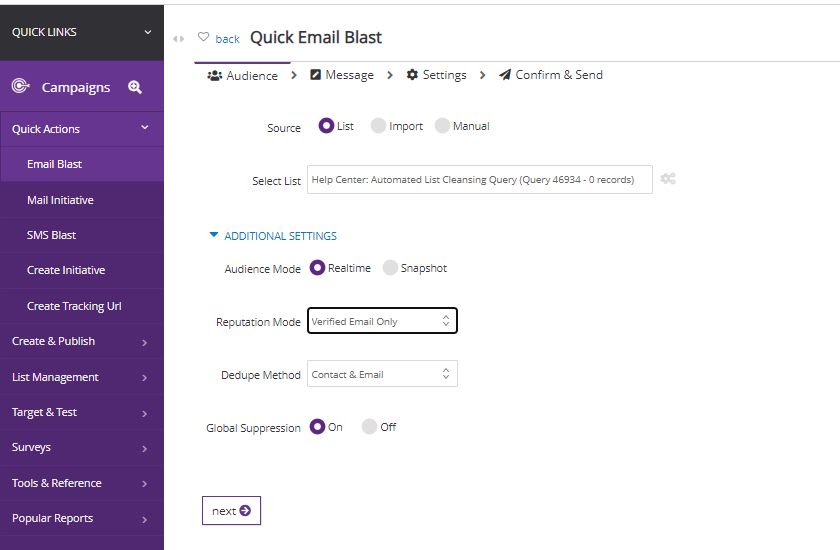The image features the user interface of the Quick Email Blast website, displaying its extensive functionalities and navigation options. On the left side, there is a vertical menu labeled 'Quick Links' at the top. This menu includes the following links: 'Campaigns,' 'Quick Actions,' 'Email Blast,' 'Mail Initiative,' 'SMS Blast,' 'Create Initiative,' 'Create Tracking URL,' 'Create and Publish,' 'List Management,' 'Target and Test,' 'Surveys,' 'Tool and Reference,' and 'Popular Reports.'

In the main content area, there are tabs labeled 'Audience,' 'Message,' 'Settings,' 'Confirm and Send,' indicating the different stages of creating an email campaign. Additionally, there are several setting options under 'Audience Mode,' including 'Real Time,' 'Snapshot,' 'Reputation Mode,' 'Verified Email Only,' and 'Dedupe Method, Contact and Email.' A 'Global Suppression' feature is also available with an on/off toggle button, currently switched to 'on.' At the bottom, there is a prominently displayed 'Next' button, allowing users to proceed to the next step in the email campaign creation process.